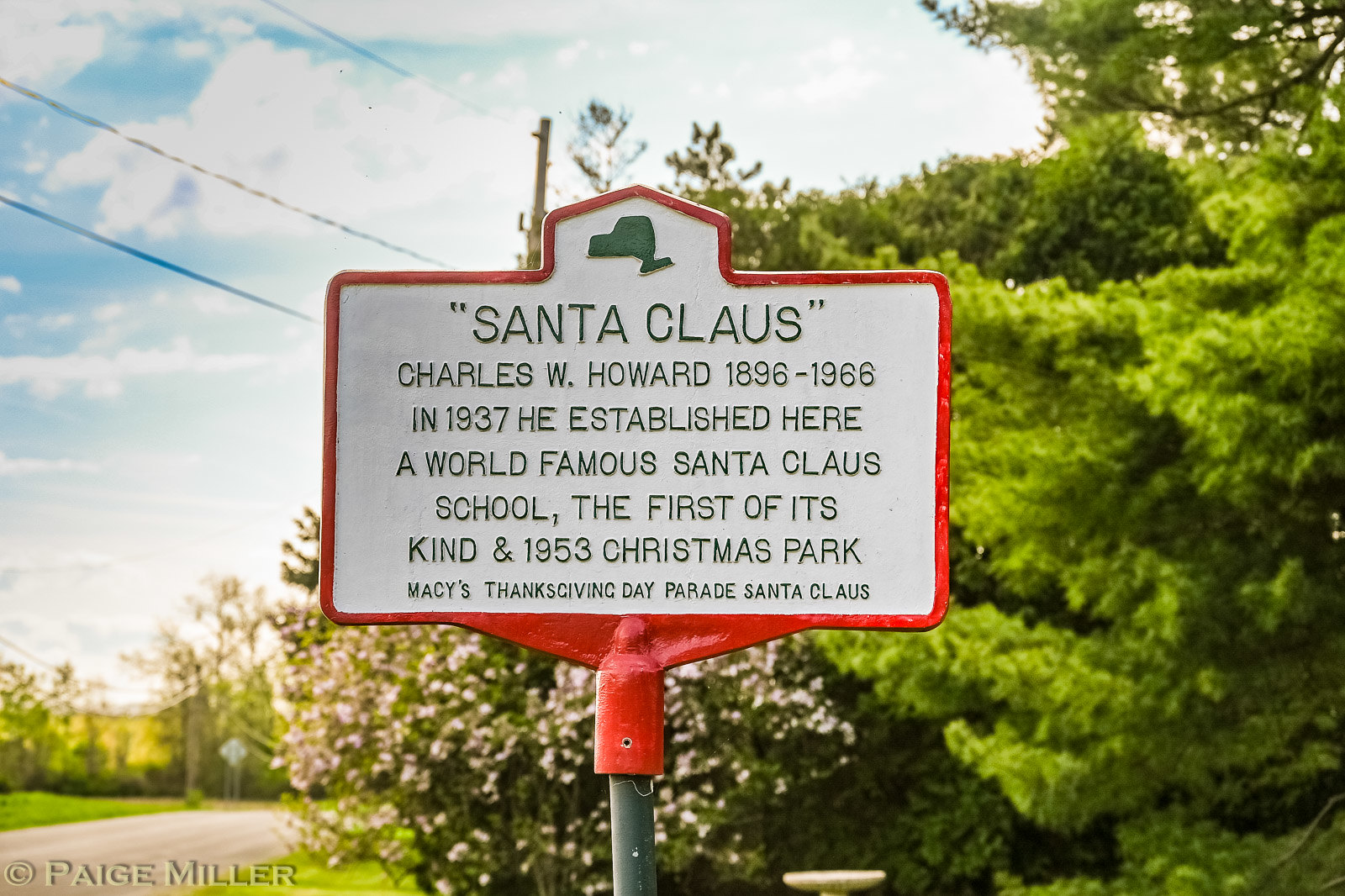The image captures an outdoor setting featuring a red-trimmed plaque mounted on a thin, silver pole. The plaque, which reads "Santa Claus" at the top in black letters, commemorates Charles W. Howard (1896-1966), who established the world-famous Santa Claus School here in 1937, the first of its kind. Beneath this, it notes the institution's evolution into Christmas Park in 1953 and mentions Howard's role as the Santa Claus for the Macy's Thanksgiving Day Parade. The background reveals a blue sky with white, puffy clouds, interspersed with some utility power lines on the upper left side. The scene also includes various trees, such as lime-green colored ones with leaves, a bush with pink flowers, and another bushy tree. In the distance, a light gray road and grassy field are visible. In the bottom left corner, there’s a transparent watermark crediting the image to Paige Miller.